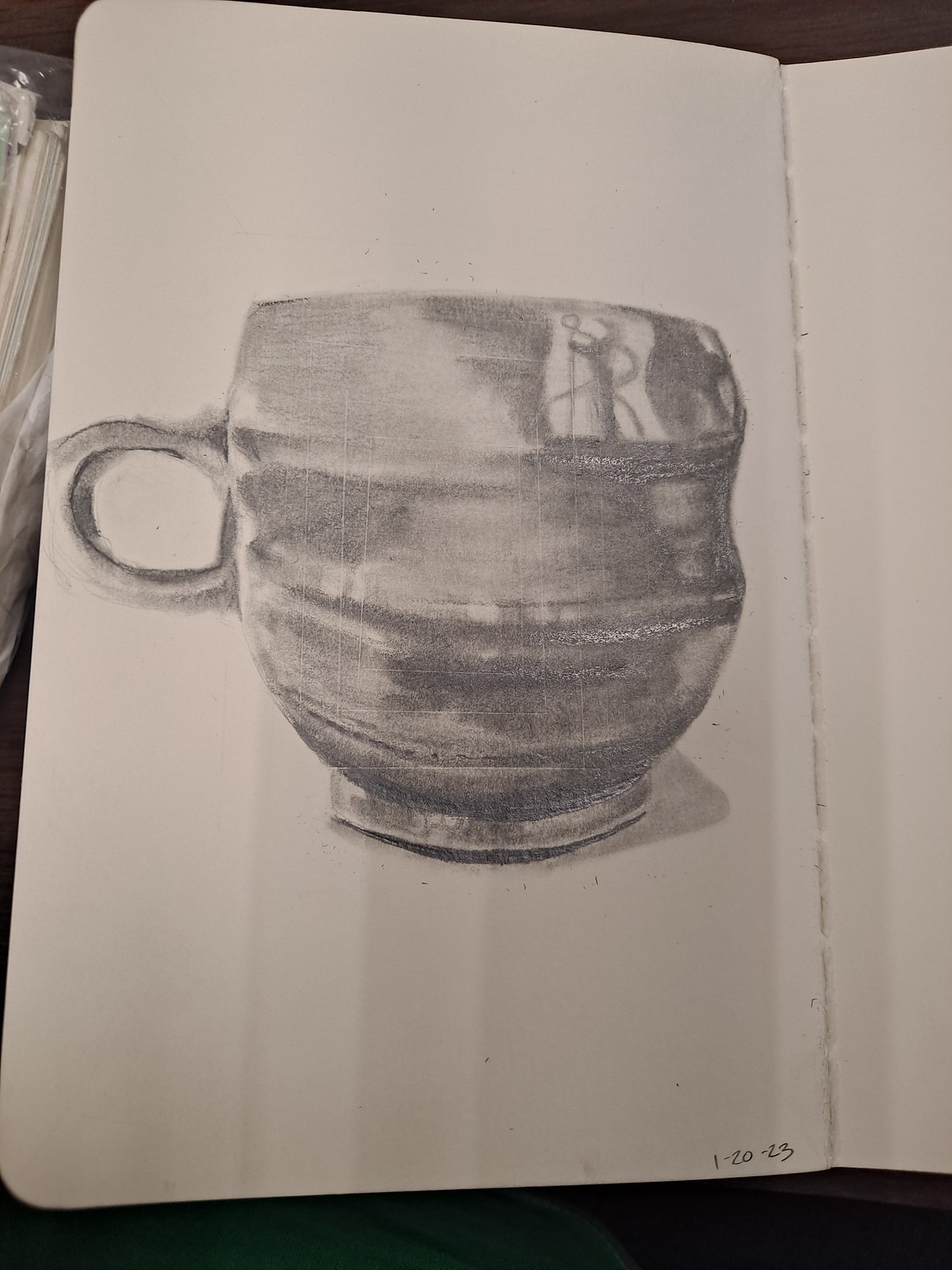A photograph captures a detailed sketch within an open sketchbook, resting on a brown table. The visible edges of the sketchbook and its central seam frame a meticulously drawn pencil illustration of a mug. The mug, positioned with its small C-shaped handle on the left, is rendered with intricate shading and highlights, suggesting a reflective surface. Surrounding the sketchbook are hints of adjacent objects, including a white item to the right. The bottom edge of the image reveals a green fabric, likely a shirt. Below the drawing, the date "1-20-23" is neatly inscribed, indicating the completion date of the artwork.